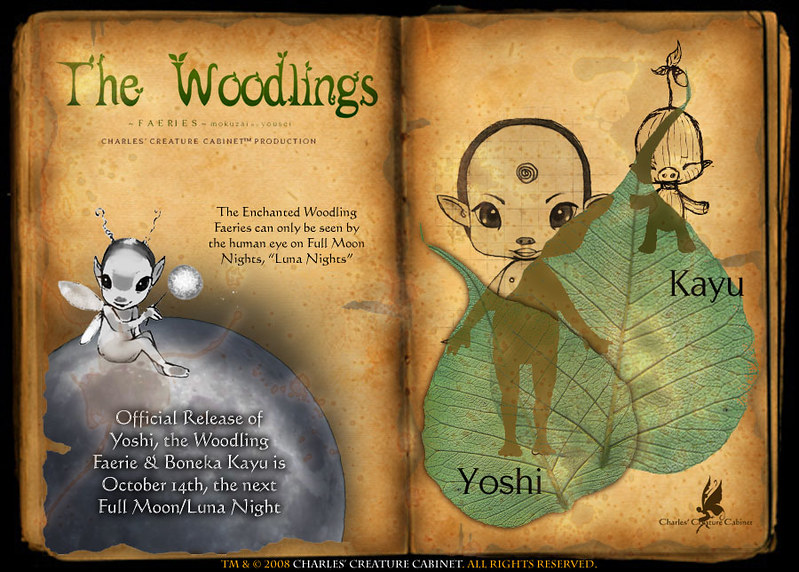The image is a digital illustration resembling two pages from an old, weathered book, set against a black background. The left page features a green title at the top, "The Woodlings," in a font resembling growing green plants. This is a Charles Creature Cabinet Production. The text explains that the enchanted woodling fairies can only be seen by the human eye on full moon nights, known as lunar nights. Below this text, there is a creature with large black eyes, pointed ears, antennae, and small wings, sitting on an orb akin to the moon. It announces the official release of Yoshi the Woodling Fairy and Boneka Caillou on October 14th, the next full moon. The right page displays two large overlapping green leaves, depicting two fairies. The one on the left, labeled Yoshi, appears more developed, while the one on the right, labeled Caillou, looks like a child version. At the bottom, the image bears the text “Trademark and Copyright 2008, Charles Creature Cabinet, All Rights Reserved.”